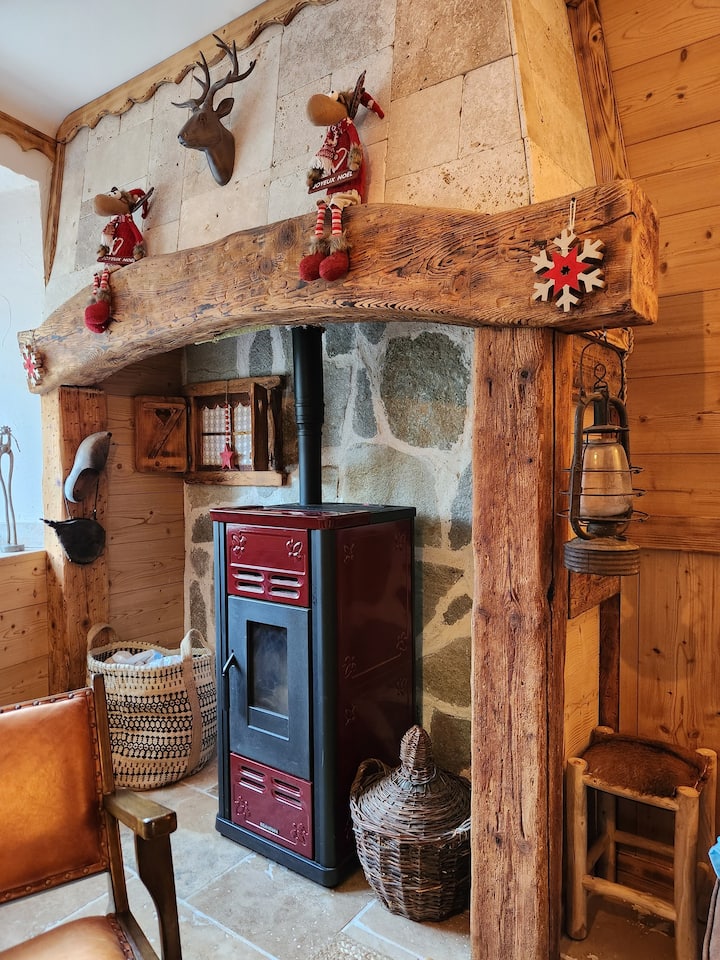In the cozy, rustic hearth of a cabin-like home, an old-fashioned, red and black metal wood stove stands where a traditional fireplace might have once been. This wood stove, with its red doors, vents, and chimney, is framed against a robust stone wall, creating a focal point of warmth and vintage charm. The area exudes a winter holiday spirit, decorated with red and white wooden snowflakes, caribou dolls, and a wooden jackalope perched above. On either side of the stove, you find practical but rustic accents: a straw basket on the floor, a large bag, and a metal kerosene lantern. A weathered wooden chair and a stool add to the inviting, cabin-like ambiance. The structure is characterized by heavy-duty wooden beams and stone floors, surrounded by wooden walls, evoking a sense of being in a Norwegian retreat. The room is bathed in bright daylight, possibly reflecting off the snowy scenery outside, enhancing its cheerful and cozy atmosphere.